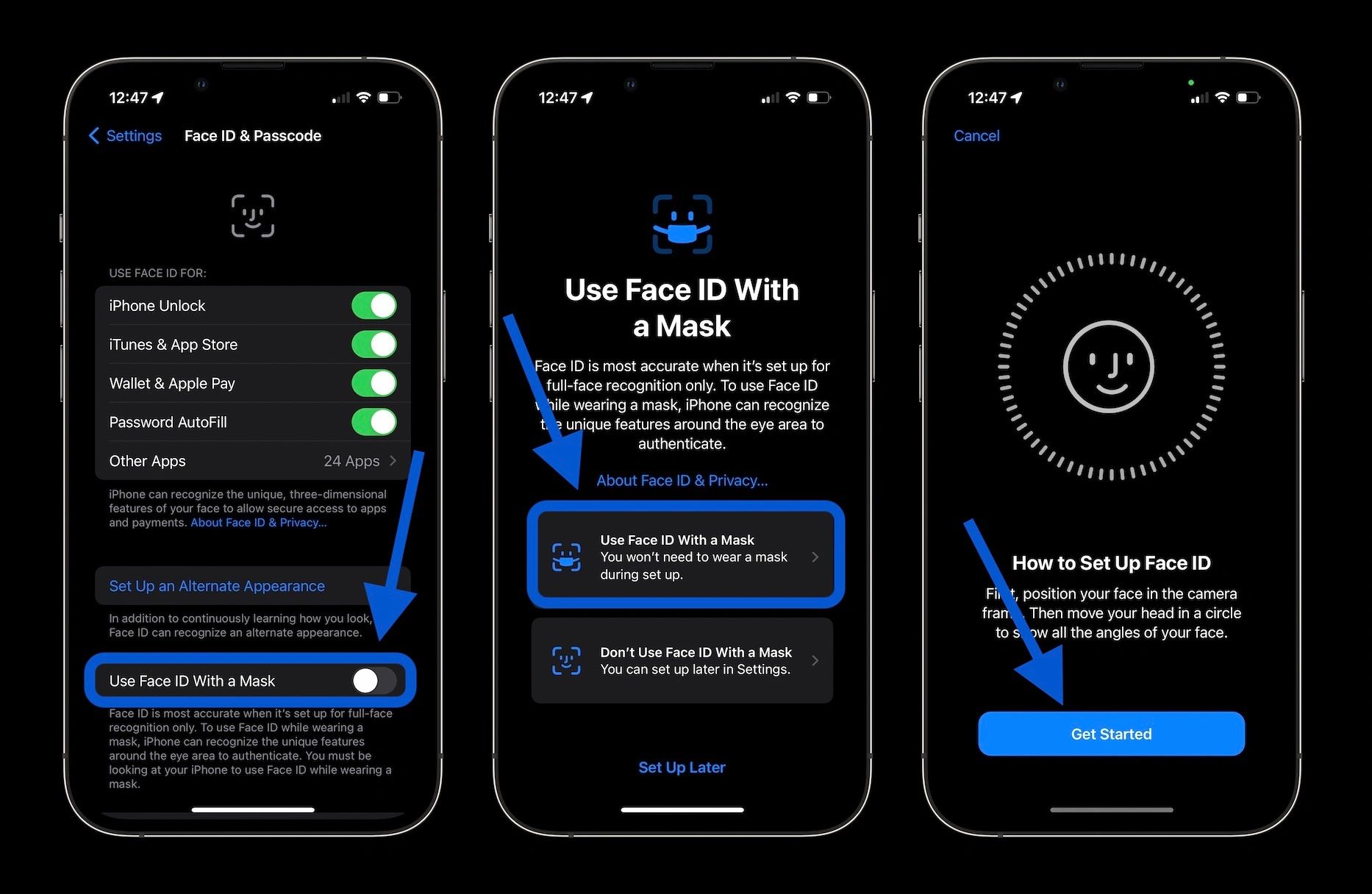This image appears to be a screenshot taken from a smartphone, depicted against a large black background. It consists of three separate screens arranged side by side, resembling the interface of a mobile device.

The first screen, located on the far left, displays a digital clock indicating the time as 12:47 in the upper left corner, next to a partially filled battery icon. The screen is open to the "Face ID & Passcode" settings, showing various options in the menu. These options include toggles for "iPhone Unlock," "iTunes & App Store," "Wallet & Apple Pay," and "Password AutoFill," all of which are turned on. Below these settings, it indicates there are settings for "Other Apps" with '24 apps' listed. A blue arrow highlights the option "Use Face ID with a Mask," which is also toggled on.

The second screen centrally features the text "Use Face ID with a Mask," and a blue arrow from the left side points towards this section. This section is highlighted in blue and includes the note: "You won't need to wear a mask during setup."

The third screen depicts the setup process for Face ID. It showcases a circular icon surrounded by small dashes and featuring a face in the middle. Directly below this icon, a blue arrow points toward a prominent blue button labeled "Get Started." Above this button, the text "How to Set Up Face ID" provides a header for the setup instructions.

Overall, this screenshot illustrates the steps and settings involved in configuring Face ID on an iPhone, with a specific focus on the option to use Face ID while wearing a mask.